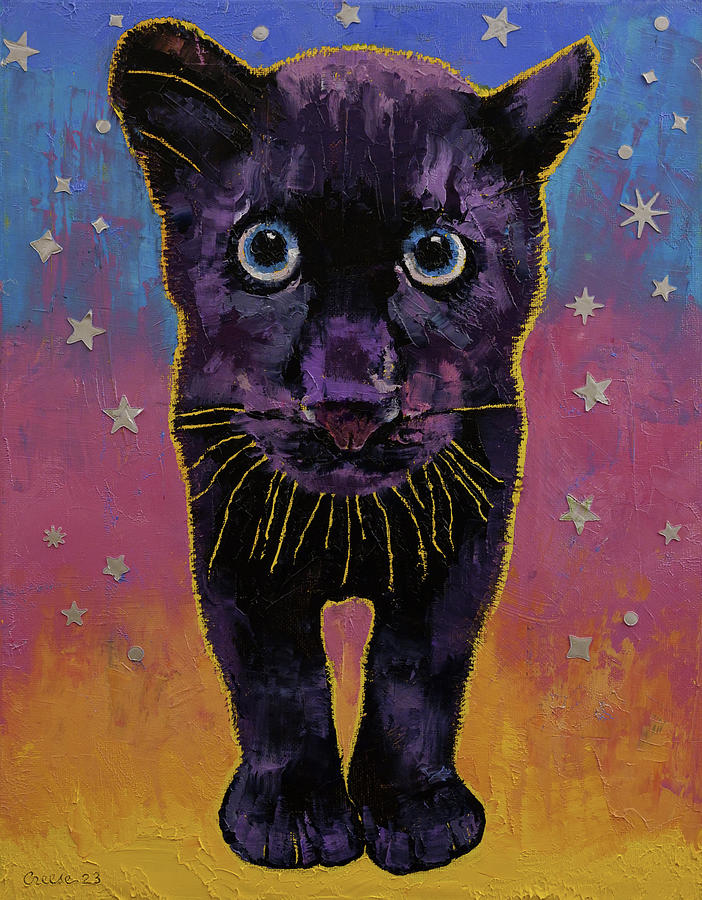This painting portrays a black panther cub with an oversized head that appears almost comically large compared to the rest of its body. The cub's face is a medley of vibrant shades—dominantly black but infused with purples, pinks, and grays, all outlined in a striking goldish-yellow color. The panther’s expressive blue eyes, with stark black centers, stare directly at the viewer, adding intensity to its gaze. The asymmetrical positioning of its ears—one facing forward, the other sideways—along with the odd depiction of whiskers around its mouth, contribute to the painting's unique, abstract character. The background features a striking gradient, transitioning from teal cerulean at the top, through pink in the middle, to orange and yellow at the bottom. Scattered across this gradient backdrop are various white cut-out shapes resembling stars and circles, adding a whimsical touch to the scene. Signed “Creese 23” in the lower left corner, this artwork has a charmingly amateurish feel that leaves viewers contemplating whether it’s the work of an emerging artist or a seasoned one employing a novel, playful style.